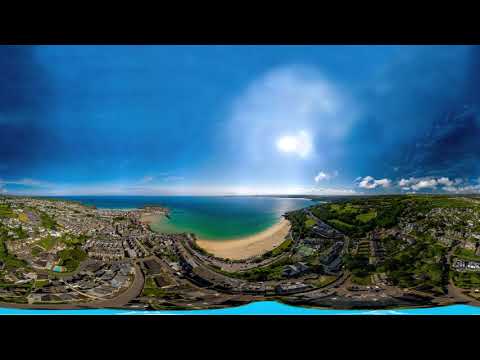This image captures a panoramic view of a coastal city, likely taken with a 360-degree lens, creating a unique, slightly distorted perspective. The photo showcases a vibrant dark blue sky, occasionally streaked with wispy clouds that congregate more densely at the bottom right. The water in the foreground transitions from a light teal near the shore to a darker blue further out, with hints of green or turquoise near the beach. A crescent-shaped sandy beach, tan in color, curves gracefully, adding to the dynamic feel of the scene. Beyond the beach, the land is dotted with abundant greenery, roads, and numerous buildings, which appear to be residential homes. Despite the wide shot and grainy quality, one can discern the layout of the city, framed by black rectangles at the top and bottom, hinting at a filter or VR effect. This busy, vibrant cityscape is encapsulated with curved streets and a verdant landscape, evoking a watercolor painting come to life.